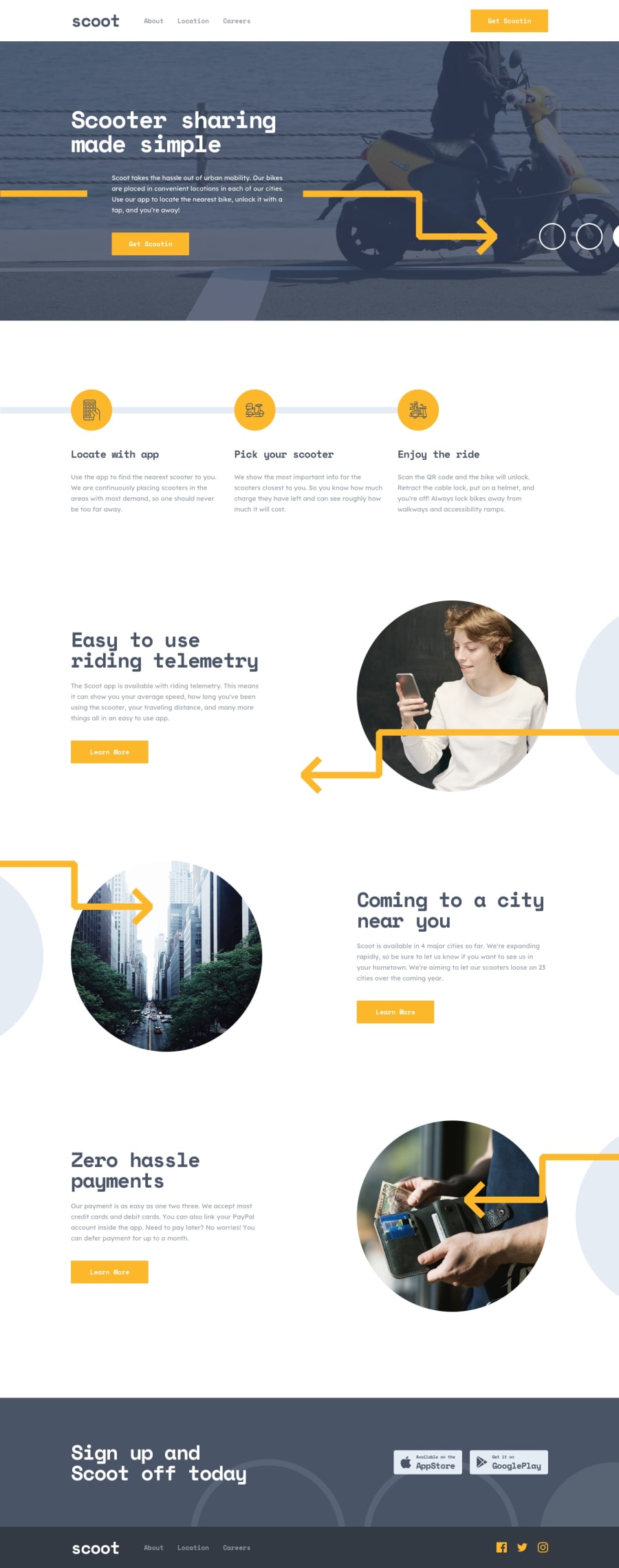The image depicts a fully zoomed-out view of the website "Scoot." At the top, the website's name is prominently displayed alongside three categories. Just to the right, there is a yellowish-orange rectangle. Below this header, the background features a gray, holographic effect with a side-view image of a person riding an electric scooter. Superimposed on this background is the tagline, "Scooter Sharing, Made Simple," accompanied by another light-orange rectangle at the bottom of this section.

Further down, there are three orange circles, each paired with corresponding text. Below these circles, the phrase "Easy-to-Use Riding Telemetry" is displayed, followed by a concise paragraph of descriptive text and another orange rectangle. To the right of this section, there is a circular image featuring a person in a white shirt using a smartphone. An orange arrow extends from the right side of this picture, curves downward, and points back to the left.

Continuing downward, there's another circular image with the caption, "Coming to a City Near You," along with the recurring orange rectangle. The bottommost part of the page declares, "Zero Hassle Payments," and includes another profile picture to the right. Finally, at the very bottom, the call-to-action reads, "Sign Up and Scoot Off Today," with two interactive tabs positioned below.